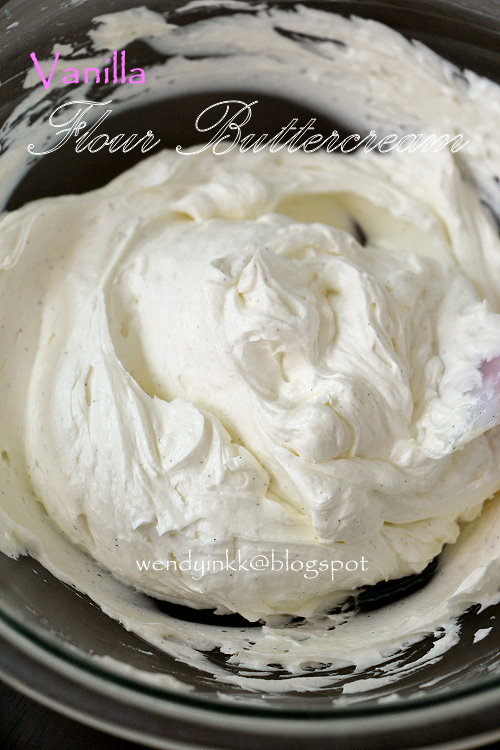The image showcases a close-up of fluffy, white vanilla buttercream frosting, heaped at the center of a black bowl with some remnants clinging to the edges. A spoon or utensil with a light pink handle is partially visible, inserted into the frosting on the right side. Distinctive text overlays the image: in hot pink font at the upper left corner, the word "Vanilla" can be seen, followed by "flour buttercream" in flowing white script. A note at the bottom in the same white font reads "WendyInkk at Blogspot," identifying the creator. The frosting appears airy and fluffy, with some vanilla bean flecks visible, although the text on the image may be somewhat hard to read due to low contrast.